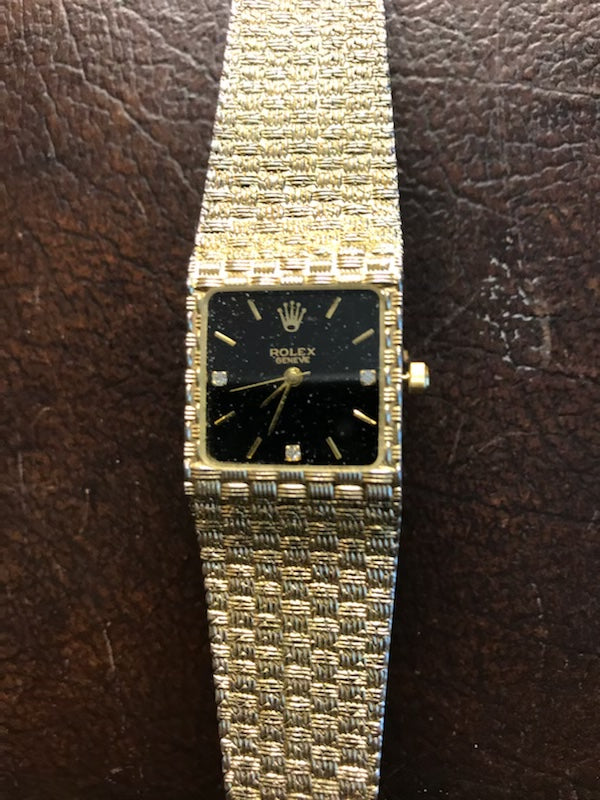This is a color photograph of a close-up Rolex watch, likely a man's model given its chunky design. The watch is laid out on a richly textured dark brown leather background, showcasing intricate grain, lines, and creases. The watch band, featuring a sophisticated woven pattern, appears predominantly gold and possibly interlaced with silver elements. The watch face is black with golden details: each hour is marked by a gold dash, except for the numbers at the 3, 6, and 9 positions which are indicated by small diamonds. The number 12 position is highlighted by the iconic gold Rolex crown logo. Centered on the watch face, beneath the crown logo, is the word "Rolex" in gold font, possibly accompanied by "Geneva". The watch hands include a second, minute, and hour hand, all set against the elegant black backdrop. The photograph, taken in portrait mode, captures the luxurious essence of the timepiece against the natural texture of leather.